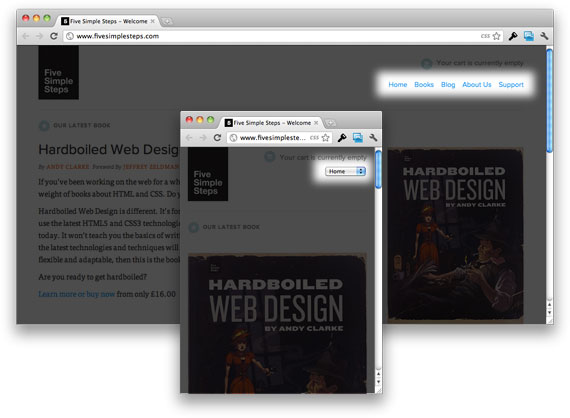The image is a detailed screen capture of a web page displayed on a Mac operating system, evident from the distinct close, minimize, and maximize buttons in the top left corner, colored red, yellow, and green. The screen capture shows a partial view of the website 'www.fivesimplesteps.com'. 

The top section of the screen features a gray header with the aforementioned colored circles on the left. Directly below this header, the site name "Five Simple Steps" is visible along with the website URL in the search bar. The main content of the image is presented in a dimmed, dark gray interface, emphasizing a highlighted section.

The highlighted segment on the right side includes a series of clickable blue buttons labeled "Home," "Books," "Blog," "About Us," and "Support." Additionally, there is a prominent image of a book cover titled "Hard-Boiled Web Design" by Andy Clark, depicting a few cartoon characters. Adjacent to this, on the left, there is a paragraph likely describing the book.

Central to the image is a secondary, vertical rectangle that extends slightly beyond the bottom of the primary capture. This inset appears to show the same web page in a more compact, minimized format, displaying only the book cover and the navigation tabs, with some sections from the main view omitted. The overall depiction is of a typical Safari browser window, characterized by its Mac user interface and organized layout.